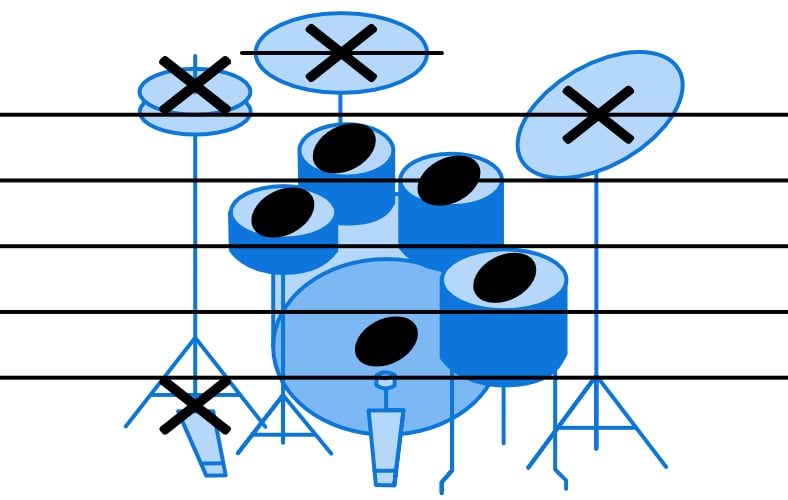This image is a detailed schematic of a typical jazz or rock drum set, beautifully illustrated in blue with varying shades for depth. The drawing includes essential elements like the bass drum on the floor, snare drums, rack toms, and multiple cymbals, each marked with an X and accompanied by a foot pedal. Horizontal black lines overlay the entire set, mimicking a musical staff complete with musical notes. These notes are strategically placed on different drums: one on the bass drum, one on the floor tom, and others on the rack toms. The precision of these elements implies a guide to where each drum note falls within a musical scale, providing both visual and functional clarity. The overall design, with its simplistic yet informative representation of circles, ovals, and lines, suggests a computer-generated origin aimed at educating or demonstrating the position and notes associated with each drum component.